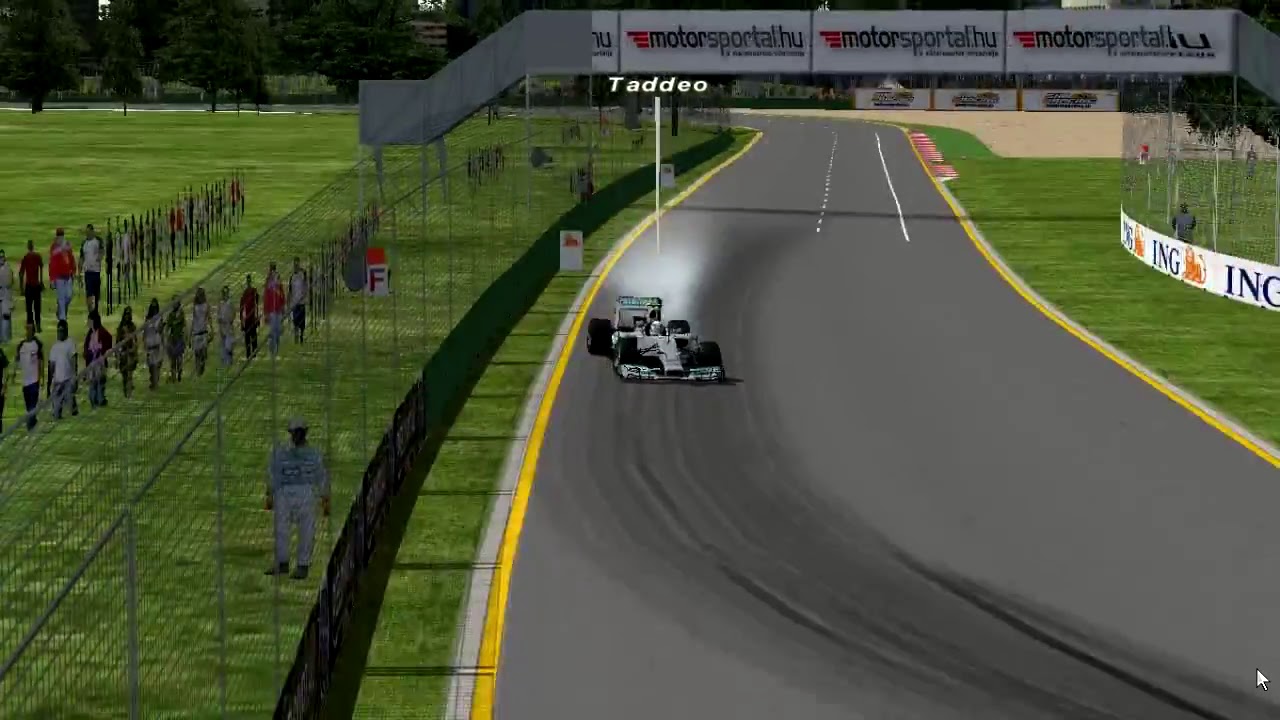The image depicts a simulated F1 race car, rendered by what appears to be video game graphics or rendering software, speeding on a paved asphalt racetrack. The race car, positioned centrally in a horizontal rectangular frame, features a white body and a green spoiler, with large black wheels, and emits white smoke as it accelerates towards the camera. The road is lined with solid yellow lines on either side, bordered by green grass. Behind a tall fence on the right, marked at the bottom with an ING banner, are rows of flat 2D cutout figures representing an audience.

Further back on the left side, a black-and-chain-link fence rises 15 feet high, and several people are visible, notably one man close to the wall and others further away. Beyond this, the scene includes trees with green leaves, expansive green lawns, and additional 2D audience figures.

White lines and red and white curbs mark the track ahead, with visible brake marks suggesting high-speed action. Overhead signage displays "Motorsport All HU," contributing to the immersive racing environment. The text "Tadeo" appears above the car with an arrow pointing to it, enhancing the interactive and dynamic feel of the image.